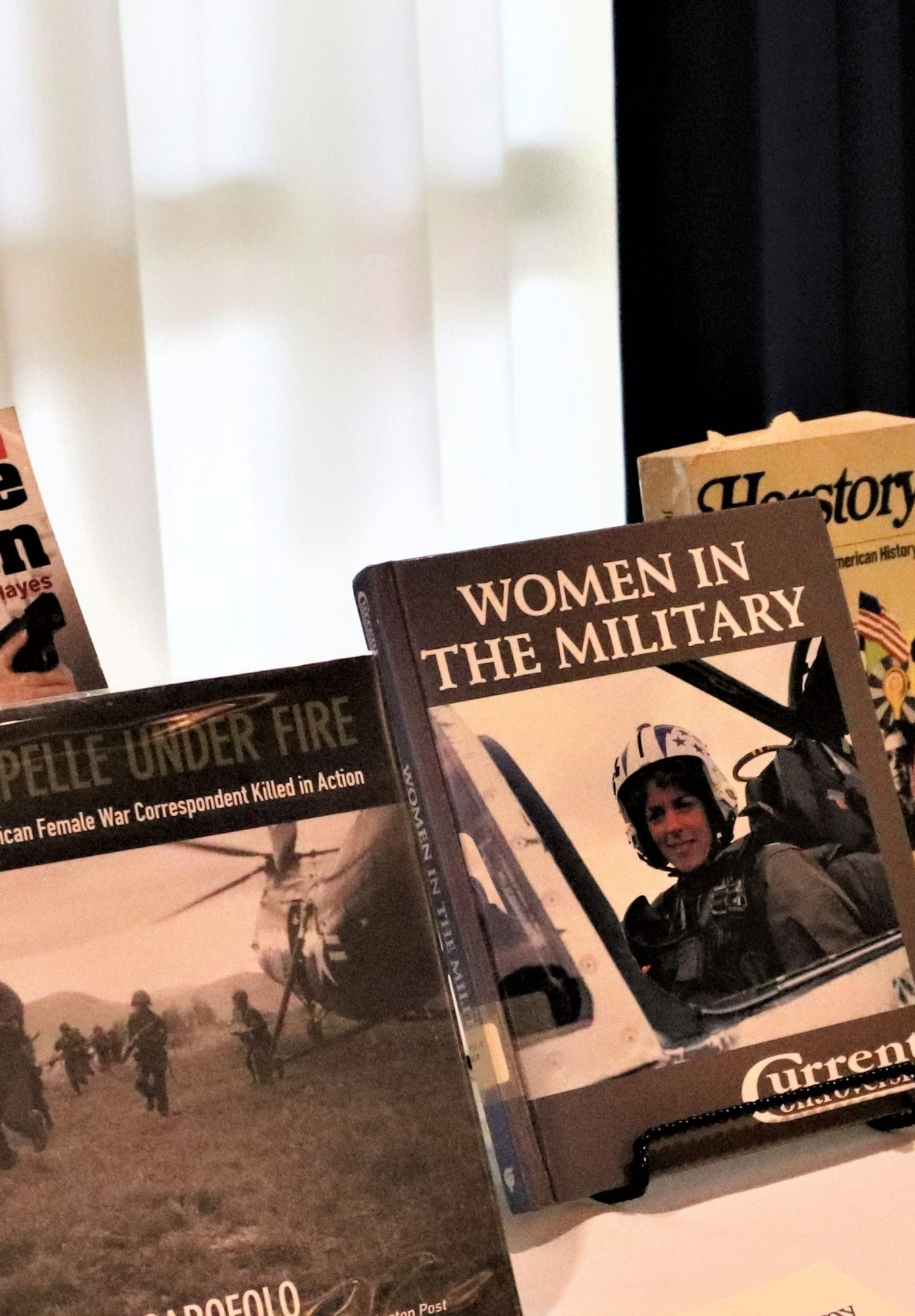The photograph showcases a collection of books artfully arranged on a window sill or adjacent table, positioned centrally at the bottom of the image. The books are stacked at an incline against a softly glowing white curtain, suggesting a light source behind it. Dominating the arrangement, the book on the far right, with a brown jacket and white text, is titled "Women in the Military." Its cover features an image of a female military pilot with dark brown hair, wearing a white helmet and a brown top. Immediately behind it is a partially visible yellow book titled "History," adorned with the United States flag. To the left, a green-titled book reads "Under Fire." There's also a barely visible book further to the left. These books, highlighting themes of military service and contributions, particularly emphasize the roles and stories of women in the military.